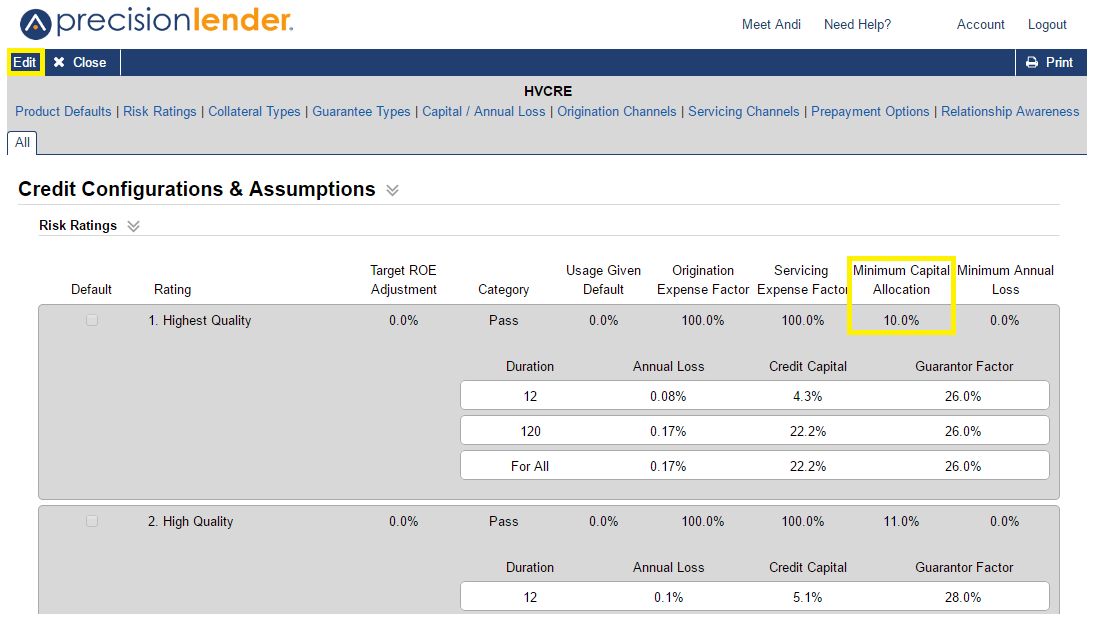The screenshot from the Precision Lender webpage prominently features an interactive diagram with various options and configurations. Across the top of the image, there are several navigational elements including "Meet ANDI", alongside options for "Need Help", "Account", and "Log Out". Just below these options, an "Edit" button is highlighted with a yellow outline, giving it the appearance of a yellow rectangle.

Centrally placed but slightly towards the right, another highlighted yellow rectangle displays the text, "Minimum Capital Allocation, 10.0%". Nearby, sections labeled "Credit Configurations and Assumptions" and "Risk Ratings" lead into a detailed list that includes options such as "Default", "Rating", and "High Quality", with corresponding checkboxes, currently unchecked. Further configurable fields include "Target ROE Adjustment", with accompanying categories of "Usage Given" and "Default".

Additionally, sections for "Origination" and "Servicing" are outlined. Toward the bottom of the image, smaller boxes contain various percentages associated with "Minimal Annual Loss". The meticulous layout of the webpage underscores its emphasis on detailed financial data and configuration settings.